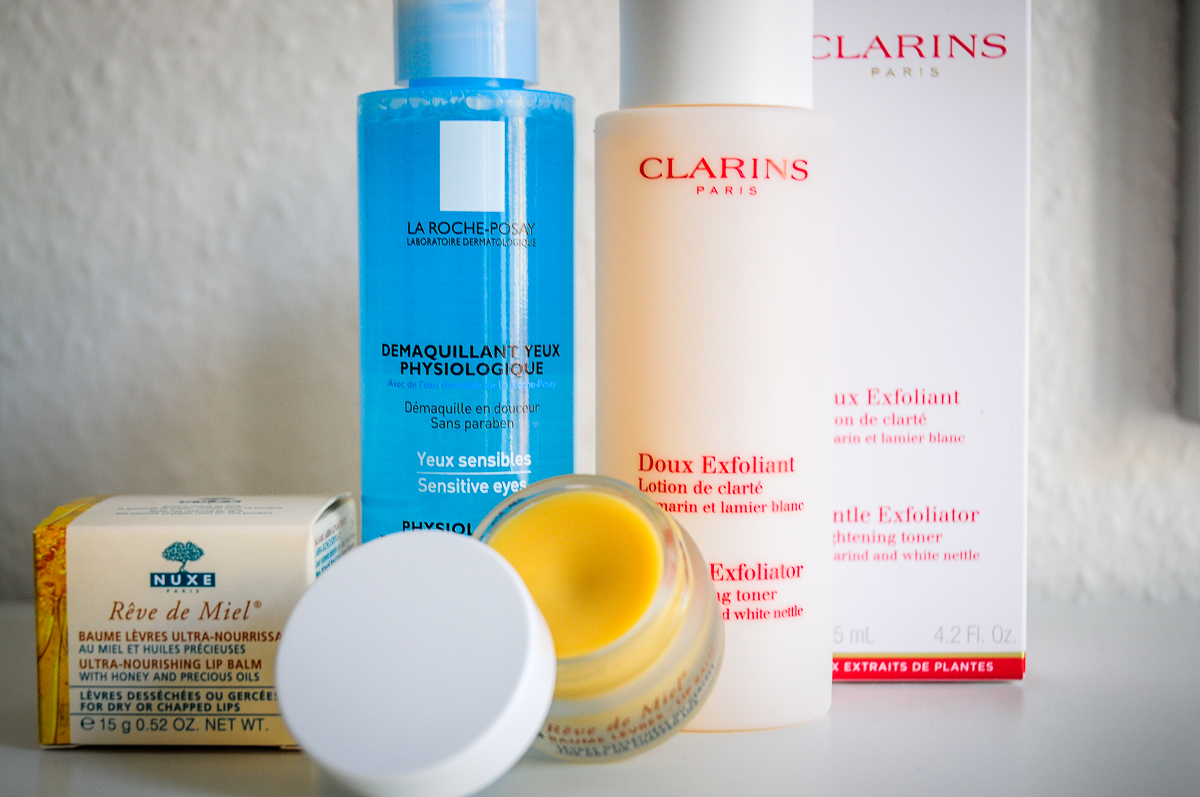The image features a textured, off-white, bumpy wall in the background. Toward the right-hand side, a small, gray window or vent breaks up the wall, marked by a darker gray horizontal line. The surface where various products are arranged is a grayish-white circular platform.

On this platform, from left to right, are several items:

1. **First item**: An orange-hued box with multiple shades of orange on the left side. It transitions into white and displays blue text on the top. The blue NUXE logo appears prominently with "Rêve de Miel" written in orange below it, including a registration mark. Smaller orange and blue text is present but too minute to decipher.

2. **Next to the box**: A clear plastic container with a blue cap, filled with a blue liquid. It features black and white text, and in front of it lies a matching white cap.

3. **Short container**: This container has an orange tone and bears writing in orange and blue.

4. **Container with a white cap**: The cap is labeled "Clarins Paris" in red. The container itself transitions from peach to white as you look from the left to the right.

5. **White box**: The box is also labeled "Clarins Paris" in red, adorned with red at the bottom, and a gold stripe above the red section.

Each product is distinct in its design, creating a visually engaging and varied composition.